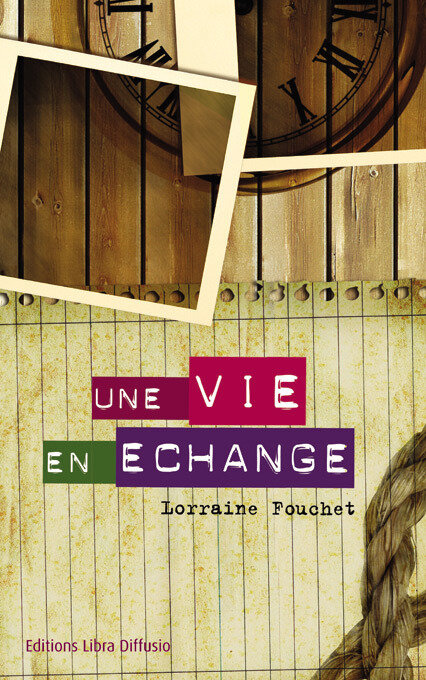The image appears to be the cover of a paperback book featuring a collage of different elements layered against a wooden background. At the top, several translucent Polaroid pictures merge to form a large clock with Roman numerals, evoking a sense of time and memory. Beneath these Polaroids, a yellowed, lined sheet of notebook paper with hole punches is prominently displayed, stained and aged. On this paper, there is text produced from a label maker reading "Un V N Echange." Below this in black font, the name "Lorraine Foucher" is clearly visible. In the lower-left corner of the image, the text "Editions Libre Diffuso" can be seen, indicating the publisher. A piece of intricately braided rope positioned diagonally in the bottom right corner further adds texture and complexity to the composition. The overall color palette includes a range of browns, tans, and other muted tones, enhancing the vintage and nostalgic aesthetic of the cover.